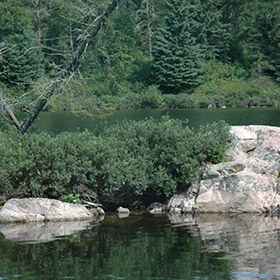This serene outdoor scene captures the tranquil beauty of a lakeside wooded area. In the foreground, calm water mirrors the lush greenery that surrounds it, complete with a couple of white-gray rocks protruding from the surface. Prominently featured is a large, vibrant green bush flanked by a small rock on the left and a larger one on the right. The reflection of this foliage in the water adds to the peaceful atmosphere. Towards the left, a dead tree trunk leans diagonally, providing a stark contrast to the verdant surroundings. In the background, the dense, wooded area boasts a variety of trees, primarily conifers and evergreens, including two distinct pine trees. The bank of this lake, possibly a river or pond, is lined with lush grasses, encapsulating the essence of nature’s tranquility.